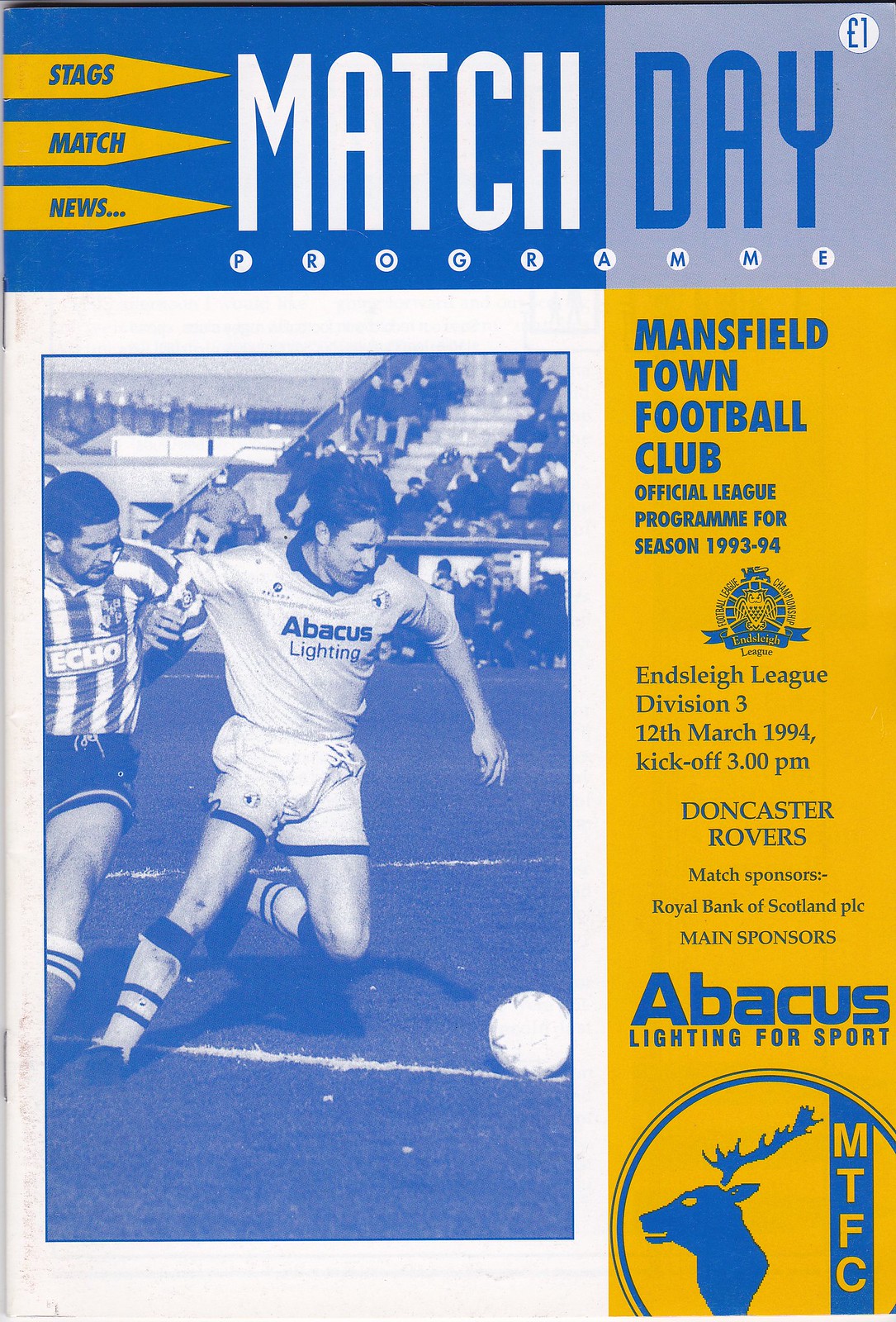The program cover for the sporting event prominently features a blue-toned photograph that spans from the bottom left corner almost to the top, depicting two soccer players vying for a ball during a game. The player to the left is wearing a shirt that says "Abacus Lighting," while the other player, donning a striped shirt that says "Echo," is jostling for the ball located to their right. The background of the lower half consists of a soccer field, transitioning to stadium stands filled with spectators in the upper half.

At the very top of the cover, a half-blue, half-light blue banner displays the text "Match Day" in contrasting white and dark blue fonts, respectively. Three stacked arrows on the left point towards the word "Match," each labeled in blue text with "Stags," "Match," and "News." On the right side, a yellow vertical banner extends from slightly below the top to the bottom, containing various informational content in blue text. 

Additional text scattered across the cover reads: "Mansfield Town Football Club, Official League Program for Season 1993-94, Ensley League Division 3, 12th March 1994, Kickoff 3pm, Doncaster Rovers." The match sponsors are listed as "Royal Bank of Scotland, PLC," and the main sponsors are "Abacus Lighting for Sport." The overall design uses a color scheme of white, blue, and gold-yellow, emphasizing the event's formal and engaging nature.